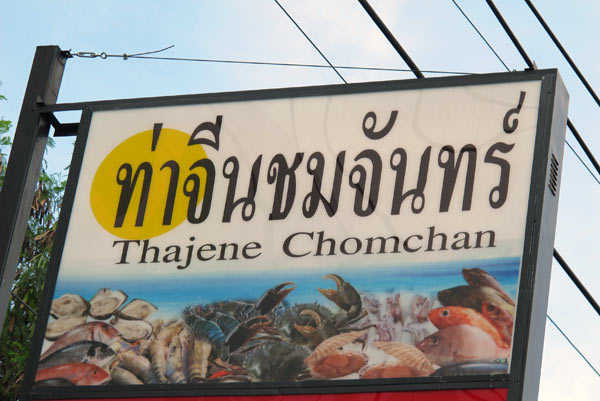This color photograph captures a horizontal sign mounted on a black pole, viewed from below against a clear daytime sky. Suspended within a black metal frame, the sign features a vibrant illustration of various seafood, including fish, crabs, and oysters, arranged on a table against a blue ocean horizon backdrop at the bottom. Above this, the top half presents a white background adorned with large black lettering in a foreign script, possibly reading "M-O-K-Y-N" or "H, O-H-N-S" over a text line stating "Daijin Chomei." Notably, the initial letter of the restaurant's name is accentuated by a golden yellow circle. Power lines and a tree are visible in the background to the left, adding to the image's urban street ambiance. The overall style of the sign is photographic representational realism, making it likely a seafood restaurant advertisement.